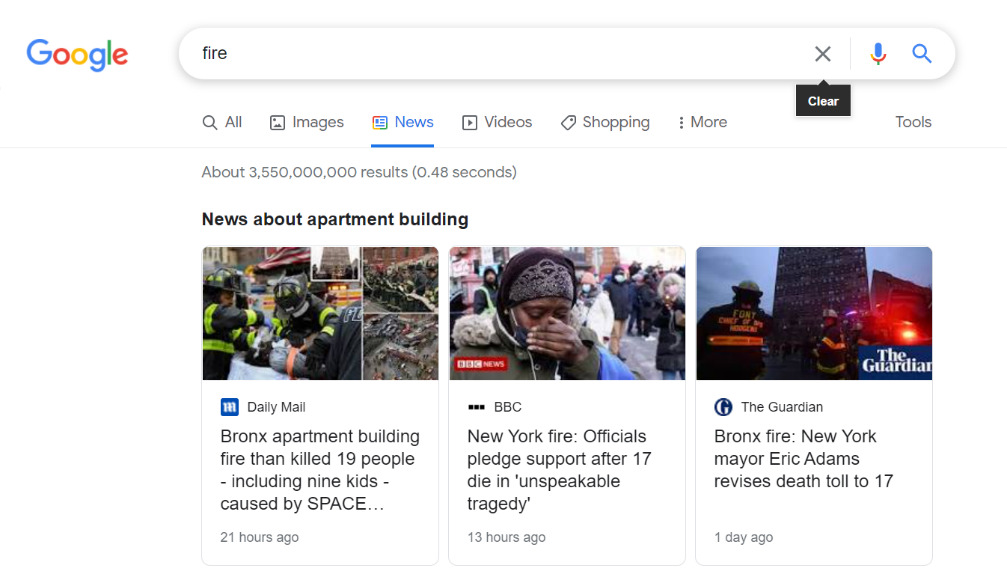This is a screenshot of the Google search results page. In the top left corner is the iconic Google logo. Adjacent to the logo, at the center of the page, is the search bar containing the query "fire." On the right end of the search bar, there is a small 'X' icon enclosed in a black square, allowing users to clear the search term. To the right of this 'X' is a microphone icon, colored blue and red, used for voice search. Next to the microphone is a blue magnifying glass icon to initiate the search.

Below the search bar, the navigation options are laid out horizontally. Aligned to the right is the "Tools" link, while the left side displays various filter options: "All," "Images," "News," "Videos," "Shopping," and "More." Beneath these filters, in gray text, is the number of search results generated.

Further down, the search results are headed by a bold headline related to recent news about apartment buildings. Under this headline, three articles are listed, each accompanied by a brief snippet of text and a relevant thumbnail image.